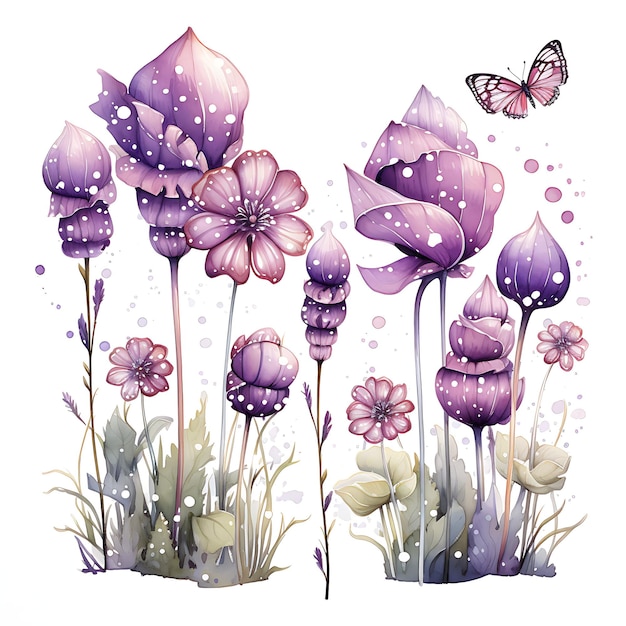This is a digital, square image with no border, set against a white background. It showcases an artistic rendering of various flowers and a butterfly, predominantly using shades of purple. The flowers vary in size, with most being fully open and decorated with intricate white dots. Among these purple blooms, some in the lower right corner are notably smaller and completely white. Green leaves and stems, punctuated by occasional pink and pinkish-yellow hues, rise from the bottom where a single, detailed flower stands out centrally. In the lower left and right corners, additional leaves and plants contribute to the natural scene. A prominent butterfly, with wings spread open in shades of purple, black, and white, occupies the upper right corner, adding dynamic movement to the composition. The watercolor-like precision of the image ensures no pigments bleed outside their contours, creating a crisp and colorful visual display.